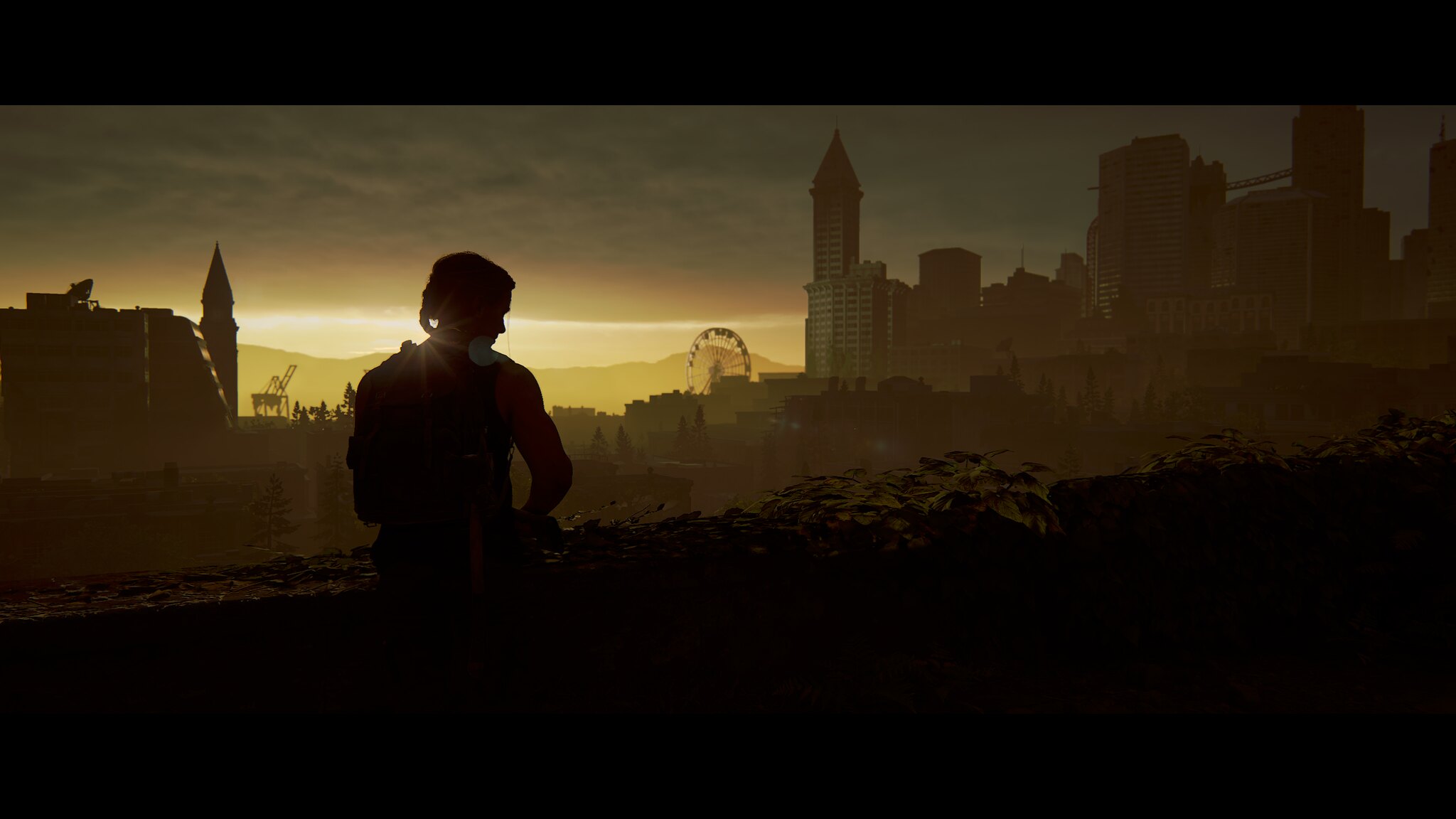In the image, which appears to be digitally rendered or heavily post-processed, a muscular figure stands on a dark ledge, silhouetted against the soft, glowing light of a sunset sky. The figure, whose gender is ambiguous, has their head turned sideways and is wearing a sleeveless vest or shirt. Their silhouette is almost completely dark, making detailed features indiscernible. The background reveals a sprawling cityscape with numerous skyscrapers and high-rise buildings. Prominently featured are a large ferris wheel and a pointed tower, possibly equipped with a satellite dish, on the left. Scattered across the scene are trees and a high-rise building, adding to the urban landscape. The sky is a captivating blend of golden yellow and yellowish-brown hues, with overcast clouds and rays of light emitting around the figure's neck, suggesting a setting sun partially obscured by their silhouette. Green leaves or foliage slightly frame the scene, enhancing the atmospheric depth of this detailed and evocative image.